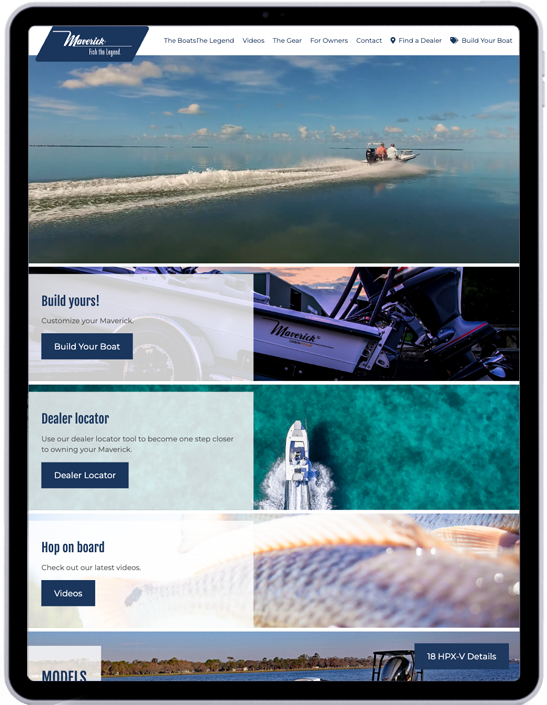The image depicts a section of a webpage or app dedicated to the Maverick boat brand. 

In the top-right corner, the name "Makik" appears in white text, although it is somewhat blurry. To the right, there are several navigation tabs written in blue against a white background. These tabs include options such as "The Boats," "The Legend," "Widows," "The Gear," "For Owners," "Contacts," "Find a Dealer," and "Build Your Boat."

Below these tabs, the centerpiece of the image features a boat traveling at high speed across the sea, leaving white waves in its wake. The sky above is a serene blue with scattered clouds.

Beneath the image of the boat, there are several sections with text. One section reads "Build Yours," "Customers," "Your Maverick," and "Build Your Boat" in blue text on a white background. Further down, there's another prompt, "Build Your Boat," written in blue and white.

To the right of the screen, a white and black boat is labeled "Maverick." Below this boat, a text block reads, "Dealer Locator: Use our dealer locator tools to become one step closer to owning your Maverick." There is a dark blue button labeled "Dealer Locator."

Further down on the right side, another white and blue boat is pictured driving through the blue sea with text stating, "Hop on Board: Check out our latest videos." This is accompanied by another button for videos.

At the bottom right, there is a section titled "Models" which features an 18-horsepower boat labeled "XV Details," acting as a clickable button.

In the top-left corner, there is the title of the webpage or app, "Maverick Fish The Legend," written in white text on a dark blue background.